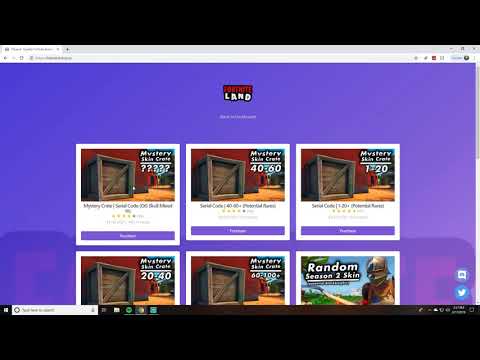This image is a cropped screenshot of the Fortnite Land website viewed on a desktop browser, set against a purple background. The screenshot is centrally positioned with a prominent black border adorning both the top and bottom edges. At the very top of the screenshot, the Fortnite Land logo is centered and scaled down, providing identity to the page. Just below this logo, there are six large white square thumbnails, each showcasing different games or templates. Below each thumbnail, a noticeable purple bar with the text "Download" is visible.

The bottom section of the screenshot reveals the desktop taskbar, featuring a search bar on the far left and several icons immediately to the right of it. Google Chrome is highlighted in the center of the taskbar, denoted by an underline, indicating it is the active application.

Lastly, at the top of the screenshot, the browser tab for the Fortnite Land page is visible, confirming the website the user is currently viewing.